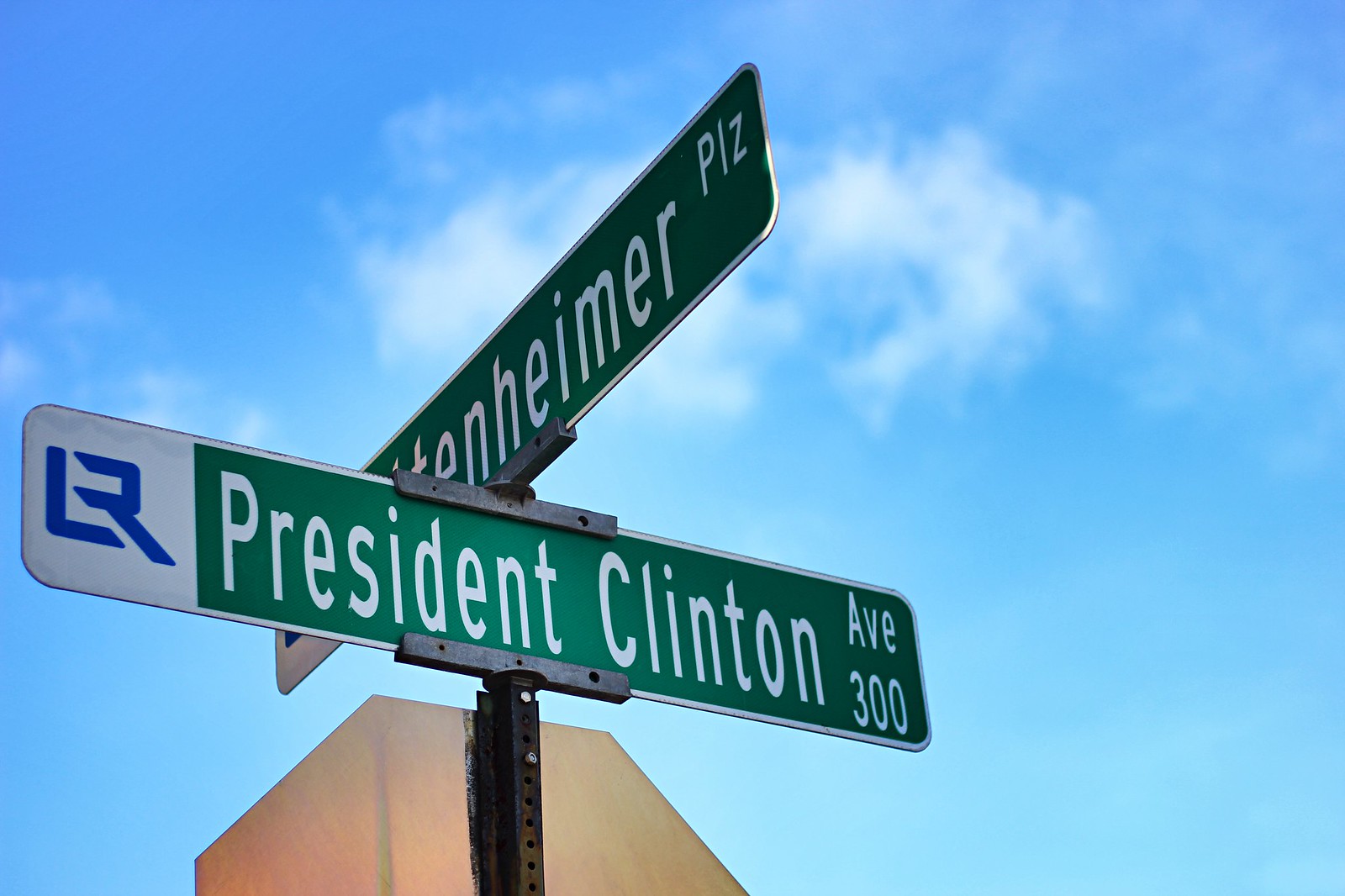The image features a street intersection, with two distinct street signs prominently displayed. The first sign indicates "President Clinton Avenue 300" in bold, clean white lettering against a vibrant green background. The second street sign, though partially obscured, reveals the name as "TENHEIMER Plaza." Both signs are long and rectangular, predominantly green with a corner section that is off-white or white. In this white section, there is a blue emblem, possibly an "R" or similar symbol, adding a unique and official touch to the design. The signs are clearly captured, providing crucial navigational information within the urban landscape they signify.